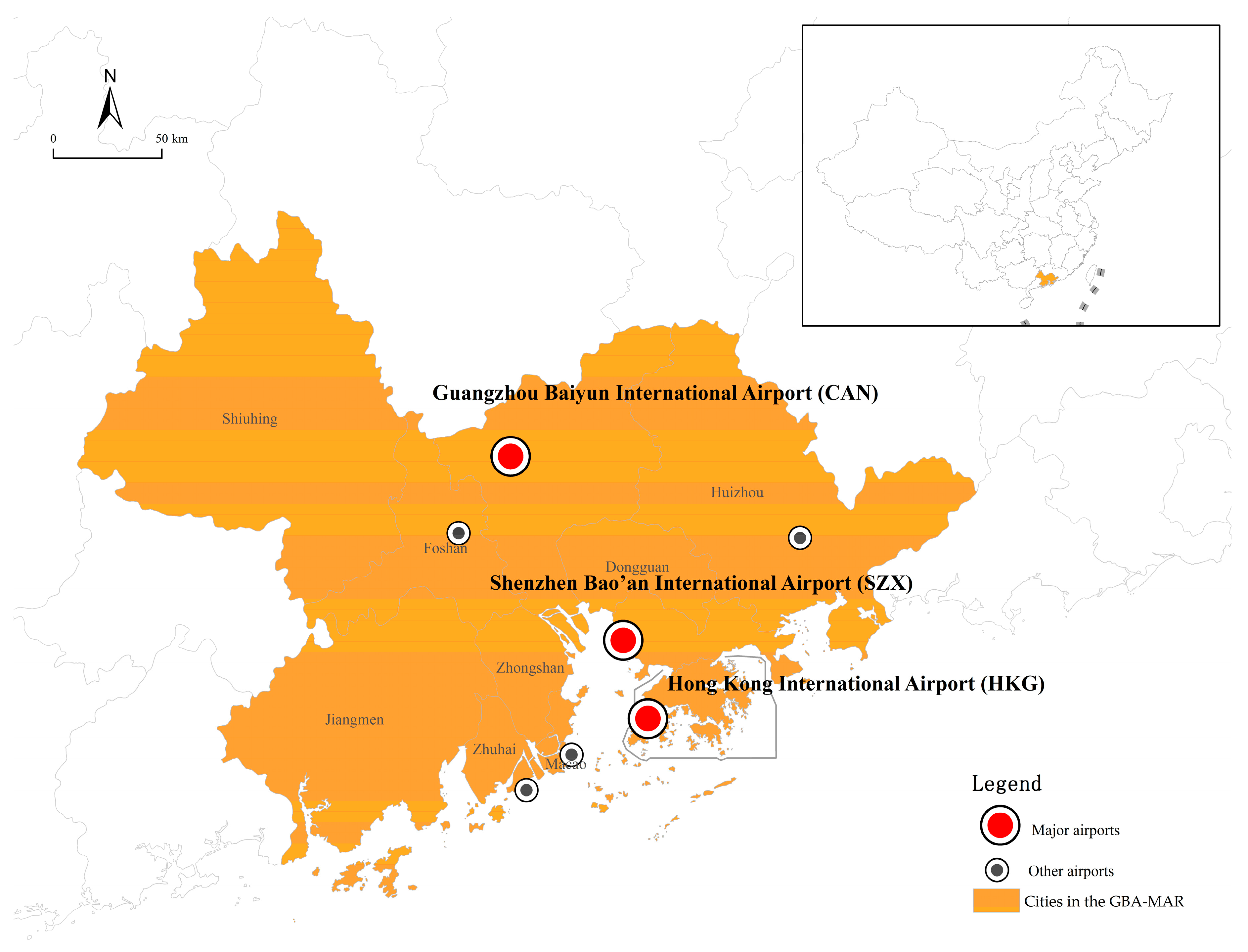The image depicts a detailed map prominently featuring a large orange-colored region representing cities in the GBA-MAR. Against a white background with thin gray outlines delineating country borders, three major airports are marked within this orange area. At the top center, Guangzhou Bayan International Airport (C-A-N) is indicated with a large circular red dot, outlined in white and black. Moving southwards, near the middle, Shenzhen Bao An International Airport (S-Z-X) is similarly marked. In the lower right, Hong Kong International Airport (H-K-G) is also denoted with the same red dot symbol. 

The map includes a legend in the lower right corner, specifying that the red dot with a black and white outline represents major airports, while smaller black circles signify other airports. Additionally, a small inset map in the upper right corner, bordered in black, highlights the large orange region within a broader context, indicating the local area targeted on the main map. Above the main map, a compass with a 'N' for north and a scale bar marking 0 to 50 kilometers provides orientation and distance measurement.